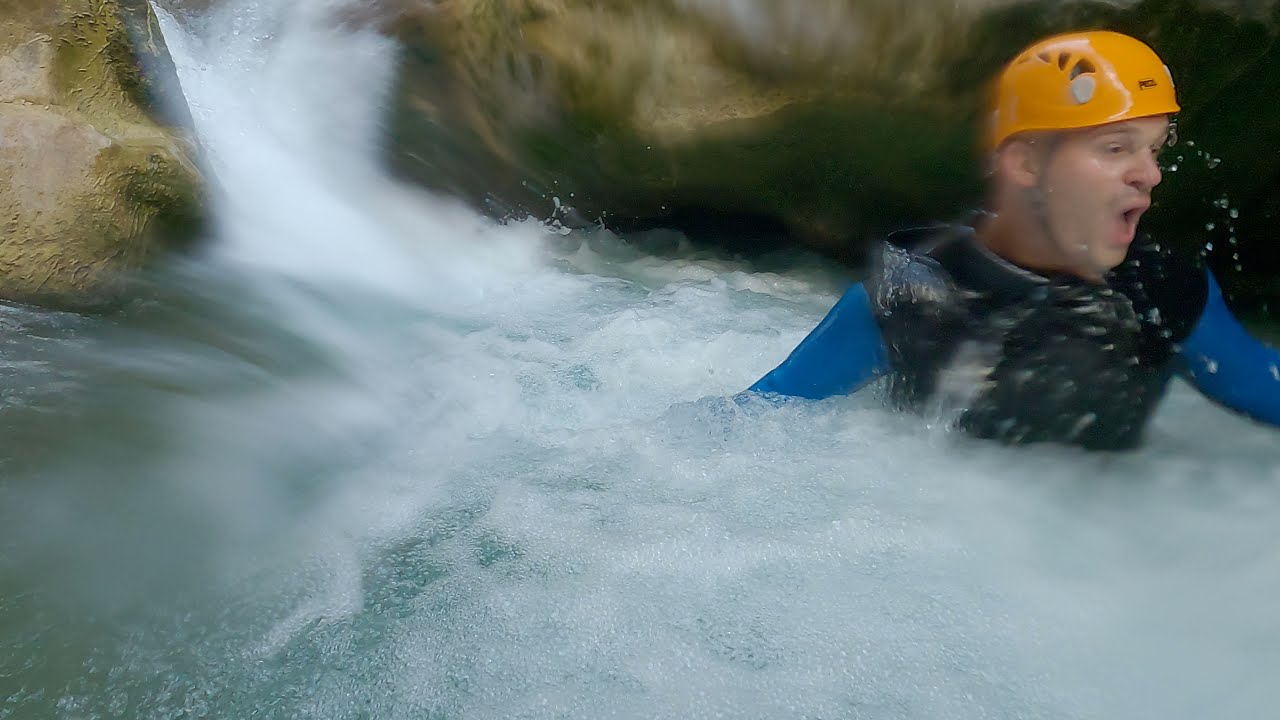The image is a rectangular, outdoor photograph, capturing the intense moment of a man engaged in a white-water rafting activity. Despite being slightly out of focus and blurry, likely due to motion and camera quality, the photograph vividly conveys the chaotic energy of the scene. The man is submerged in swiftly moving water up to his mid-chest, surrounded by white foam and turbulent currents. He is clad in typical white-water rafting gear, including a yellow helmet, a blue shirt, and a black life jacket. His expression is one of shock, with his mouth agape and eyes wide, as if he has just emerged from underwater. Behind him, the backdrop features a rocky area with water cascading down in a waterfall-like manner, adding to the dynamic and adventurous atmosphere of the setting.